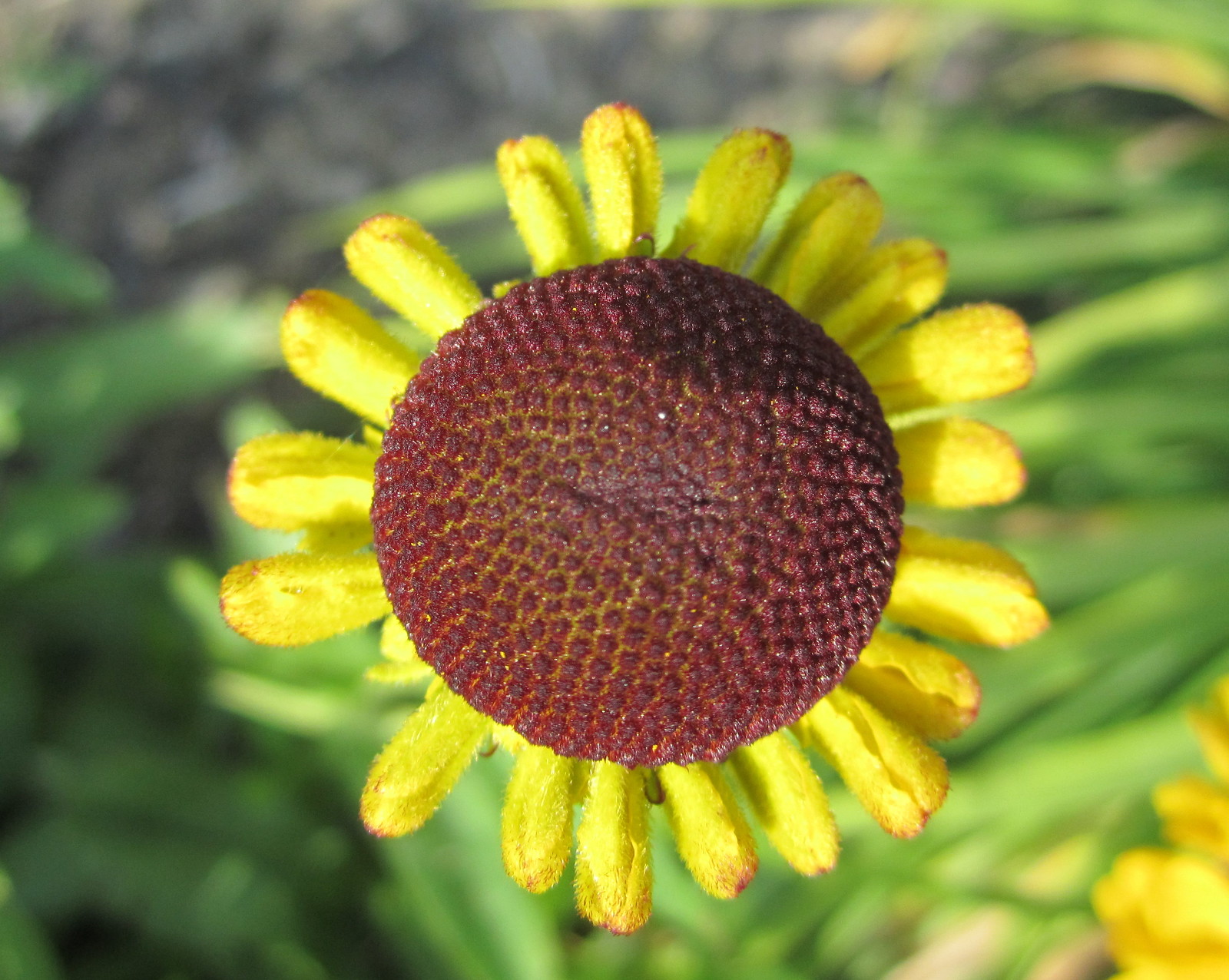This wide rectangular image captures a sunflower at the center, photographed from above, showcasing its large, greenish-brownish-reddish central disc composed of dark brown bumps. Surrounding the central disc are tiny, spaced-apart yellow petals with a fuzzy texture. The background reveals several long, blurry green leaves concentrated mostly in the top right, extending down to the left, and a few additional blurry yellow petals in the bottom right corner. There is also a notable gray area starting from the top left of the image. The sunflower appears to be beginning to wilt, suggesting the image was taken outdoors, perhaps in a garden or a farm, on a sunny day, evident from the bright and clear conditions.